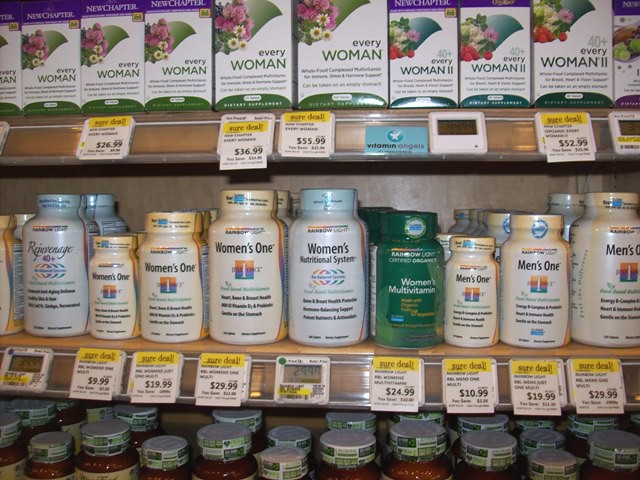This photograph depicts a section of store shelves specifically dedicated to multivitamins, highlighting gender-specific products. The display consists of three shelves, each featuring a selection of vitamins and dietary supplements.

On the top shelf, boxed items from the brand New Chapter are prominently displayed. These include products named Every Woman and varieties such as 40 Plus Every Woman 2. The packaging is primarily green, and the boxes are accompanied by price tags, with notable prices being $26.99, $36.99, and $55.99. Additionally, there are promotional tags labeled "sure deal" and a small blue label indicating "Vitamin Angels."

The middle shelf contains various bottles of supplements, including brands like Women's One, Women's Nutritional System, and Men's One. The Women's One and Women's Nutritional System bottles are visibly light orange and blue, while another bottle is green and labeled Women's Multivitamin. Different sizes and types of Men's One supplements are also present. Prices here range from $9.99 to $29.99, with several price tags displaying amounts such as $10.99, $19.99, and $24.99.

The bottom shelf is partially visible, mainly showing the caps of vitamin bottles. These caps are white with green and clear plastic seals, though the labels on the bottles are not fully visible. The photo cuts off at this point, making it difficult to discern the specific products on this shelf.

Overall, the shelves showcase a wide array of gender-specific multivitamins, with detailed pricing and a mix of bottles and boxed items.